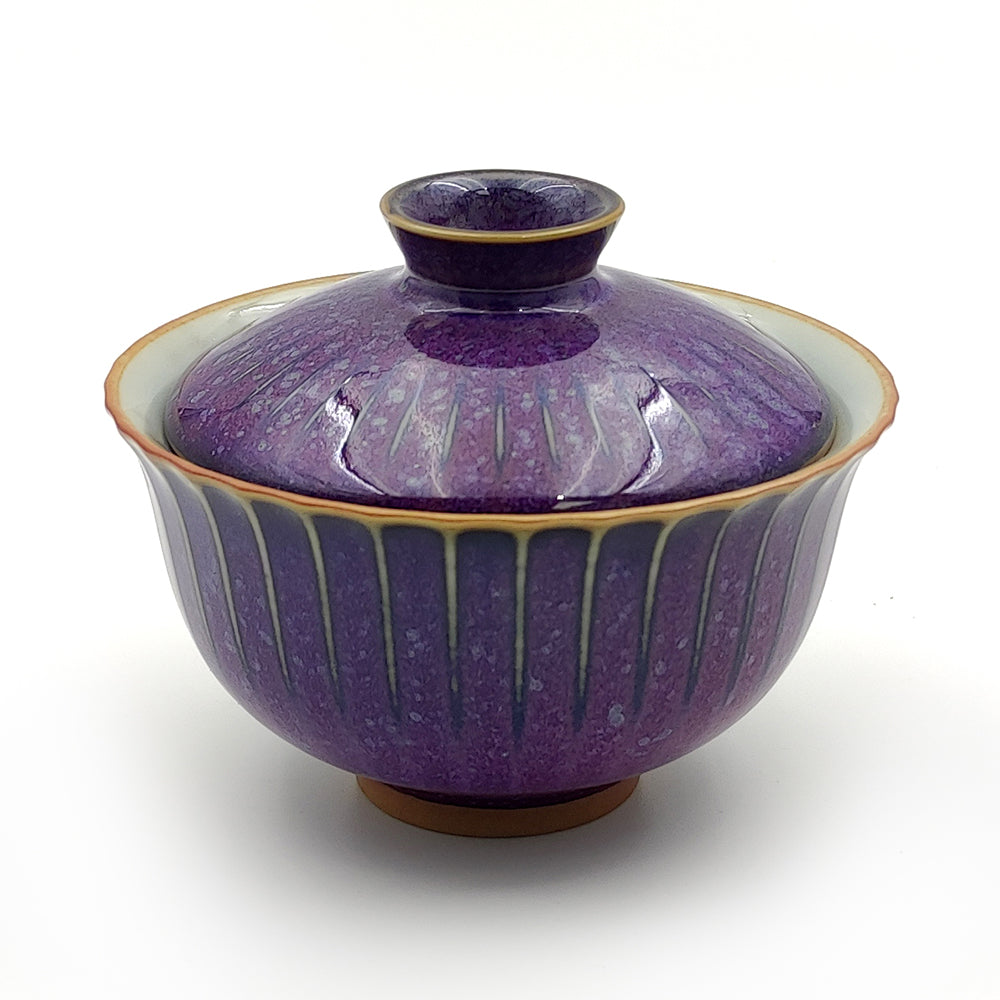This photograph showcases an elegant piece of glazed ceramic dishware, featuring a high-walled, purplish bowl with a lid. The purple hue of the bowl is accentuated by tapered beige lines that extend from the top rim and taper downwards, creating a striking visual effect. The bowl stands on a small, brown terracotta ring, providing a sturdy base. The exterior of the bowl includes a drippage design that adds to its artisanal charm, while the interior is a contrasting white, offering a clean, bright look.

The lid fits snugly, sinking about an inch into the bowl's lip. It is dome-shaped with a small circular handle on top, designed to mirror the bowl's aesthetic with the same purple and beige detailing. The lid features tiny oval-like beige accents arranged in a manner that mimics slits but are, in fact, decorative patterns. Both bowl and lid share a glossy, shiny finish that enhances their sophisticated appeal.